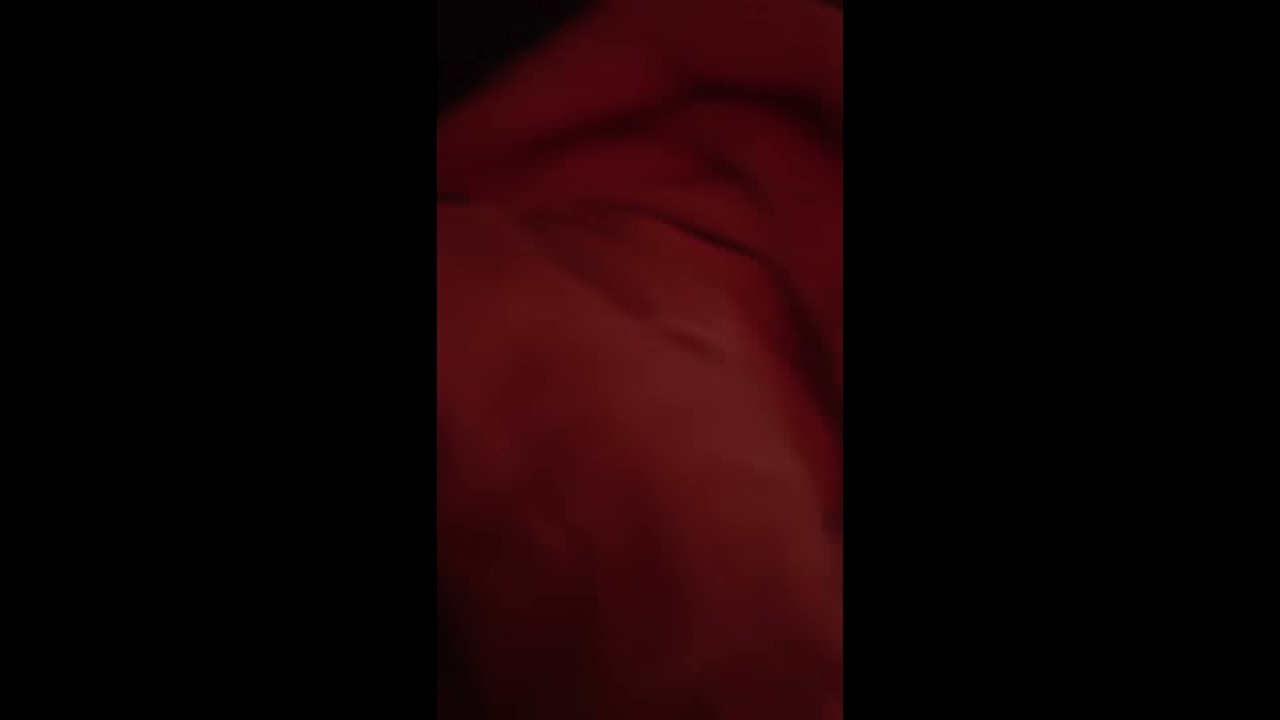This image is a close-up, color photograph in portrait orientation, set against a solid black landscape-oriented background. The central image, captured in dark red tones with varying shades of gray, depicts a highly zoomed-in section of a person's face, specifically focusing on an eyebrow, the closed eyelid below it, and part of the person's nose and cheekbones to the right. The arching eyebrow is dark brown in color, and below it, the eyelid is devoid of eyelashes. The top part of the nose is visible, with the nostril peeking into the center-right of the frame. The cheekbones flow toward the right, adding to the subtle texture and depth of the photo. The top left corner of the image is a solid black, enhancing the dramatic contrast. In its play of shadows and highlights, the image leans towards abstract photographic representationalism, creating an effect that could resemble natural landscape features or textured material, such as rumpled red bedsheets.